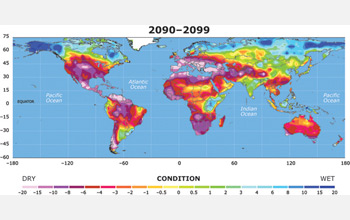This image is a detailed topographic map of the Earth, presented on a flat background, indicating global climatic conditions for the period from 2090 to 2099. The map spans from the United States and South America on the west to Australia on the east, also depicting the Pacific and Atlantic Oceans, as well as continents like Asia, Russia, and Africa. The map is overlaid with a color scale underneath it, labeled "condition," which measures precipitation levels. The scale ranges from dry (represented by values such as minus twenty-five) on the left to wet (plus twenty-five) on the right, with zero in the center. The colors shown include gray, purple, yellow, green, light blue, and dark blue, which are mapped across the landmasses to indicate varying degrees of wetness. Specific details, such as text and numbers, are difficult to read due to the small size of the image.